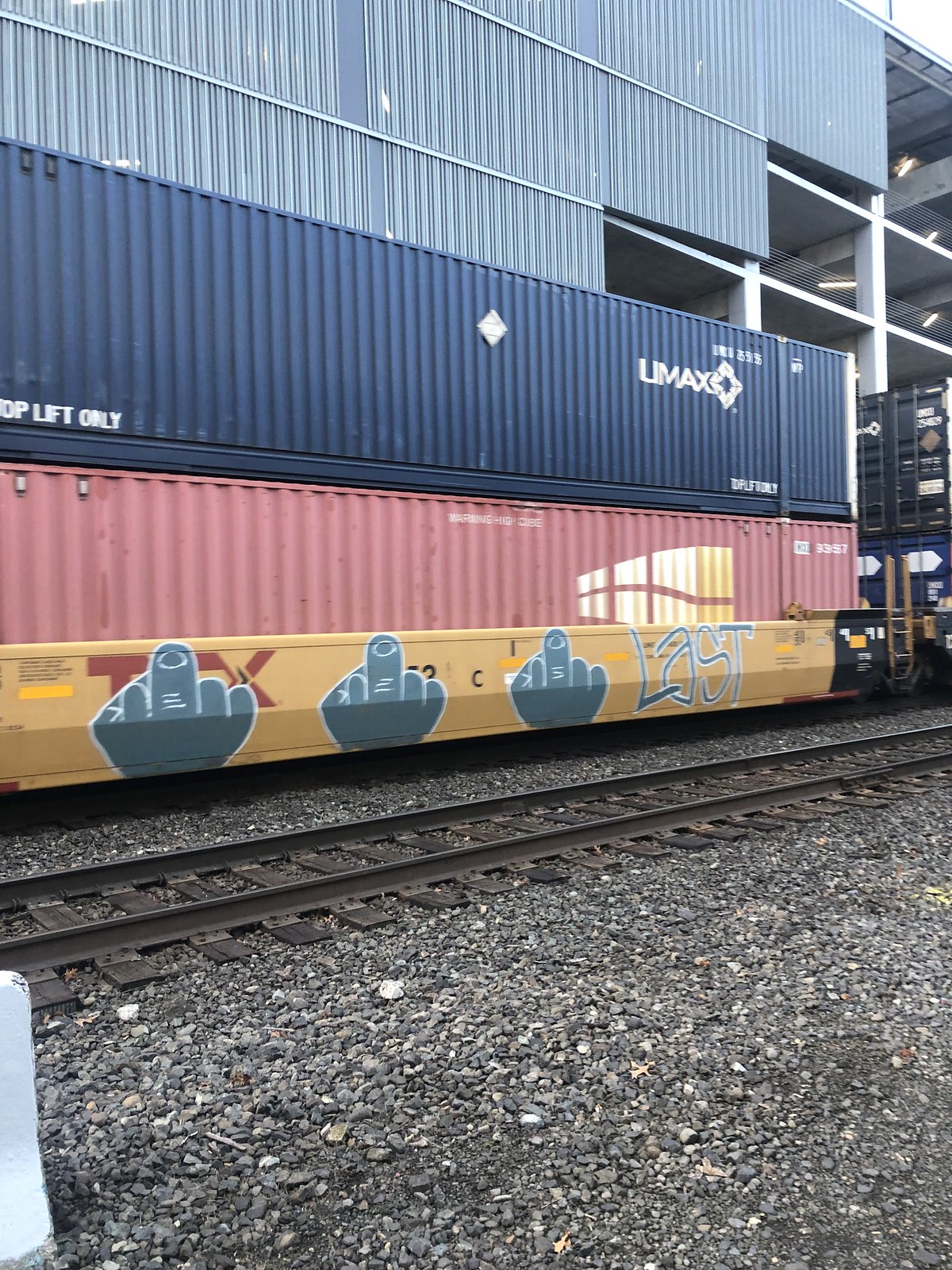This detailed color photograph depicts an urban train yard scene. The foreground reveals a gravelly ground composed of gray pebbled stones. A set of railway tracks crosses from left to right diagonally, intersecting the center of the image. The railway tracks, with their brown metal rails and wooden slats, cradle a train car of particular interest.

The train car itself is a flatbed, painted yellow, and bears distinct graffiti art. This graffiti features three large, gray, cartoonized hands each extending the middle finger, painted side by side. Next to the hands, the word "LAST" is spray-painted in capital letters. 

Stacked on the flatbed train car are two international cargo containers. The upper container is a dark navy blue, marked with the text "UMACS" in white, alongside a diamond pattern. The text "TOPLIFT ONLY" is also printed in white on either end. The container beneath it is a weathered red color, showing some white writing possibly indicating a container number, and a partly readable warning phrase. 

In the backdrop, an industrial building or parking structure with metallic paneling is visible. This building features vertical seams of standing seam paneling, transitioning from pinkish salmon in the middle section to dark blue at the top, and gray towards the bottom. Additionally, yellow illustrations and white bars appear on the building's facade. 

Loose gravel surrounds the railway tracks and the space between the stacked cargo containers. This comprehensive scene encapsulates the gritty, utilitarian aspect of an urban train yard, enriched with expressive street art and industrial architecture.